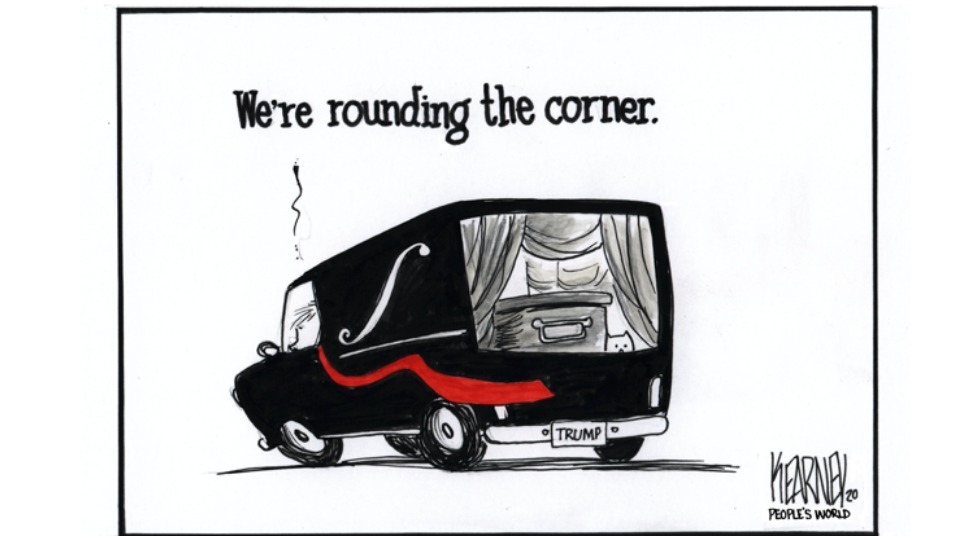This detailed description focuses on the communal details observed in the image:

The image is a political cartoon, artistically presented in a style reminiscent of a comic strip you might find in a newspaper. Dominated by a black and white color scheme with accents of red and gray, the central figure is a black hearse, viewed from a diagonal angle, slightly off-center but near the middle of the composition. The hearse bears a significant license plate reading "TRUMP" in bold black letters. 

The vehicle, which initially may appear like a van, carries an implication towards former President Donald Trump, as inferred from the license plate and the political context. Inside the hearse, a gray casket is visible, and curtains in the back hint at a small figure, perhaps a cat or dog, peeking out. 

A person is driving the hearse, which has a distinctive insignia on its left side and a prominent red stripe. Above the image, the text reads "We’re rounding the corner," suggesting a political message or commentary. In the bottom right corner, the signature "Kearney, People's World" stamps the cartoon, confirming its editorial and artistic origins.